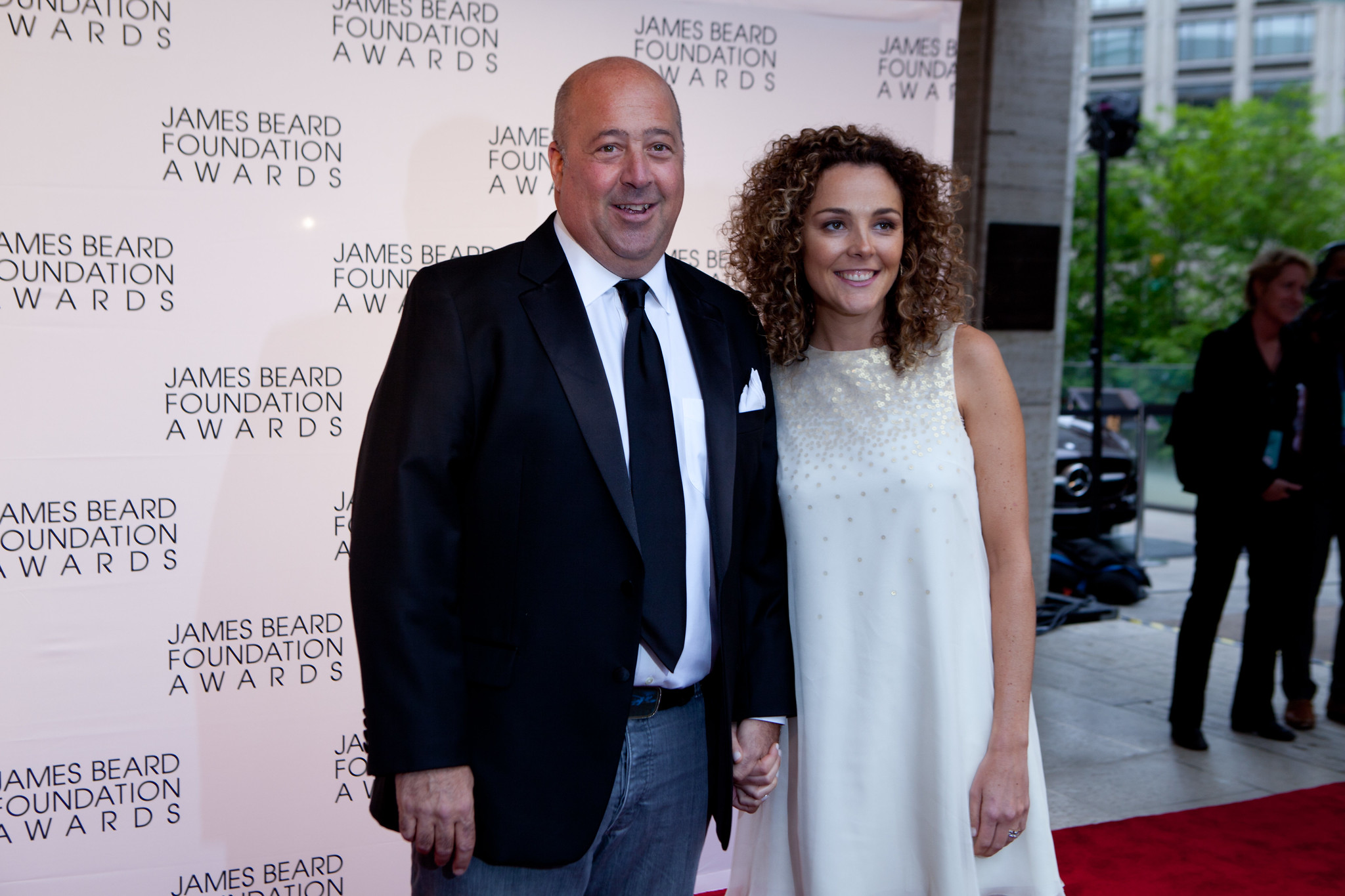This is a wide rectangular photograph of a couple attending the James Beard Foundation Awards. They are centered in the image, standing on a red carpet that only appears in the bottom right corner, starting just above and then tilting down diagonally to the left. The man on the left is fairly bulky, with tan white skin and a bald head. He smiles, showing his front teeth, and wears a white button-up shirt, a black tie, and a black blazer paired with blue jeans and a black belt. To his right stands a woman with light skin and very curly brown hair with blonde highlights. She is dressed in a sleeveless white gown that flares from the neck and features pearly colored sequins around the neckline. 

Behind them is a white banner that repeatedly reads "James Beard Foundation Awards" in black text. The setting is outdoors, as indicated by the presence of trees, a car on the street, and other people in the background, including a woman in a white dress and another man in a dark blazer with a handkerchief, near a tree and marble floor. Towards the right of the photo, part of a building with glass windows and a lighting structure is visible.